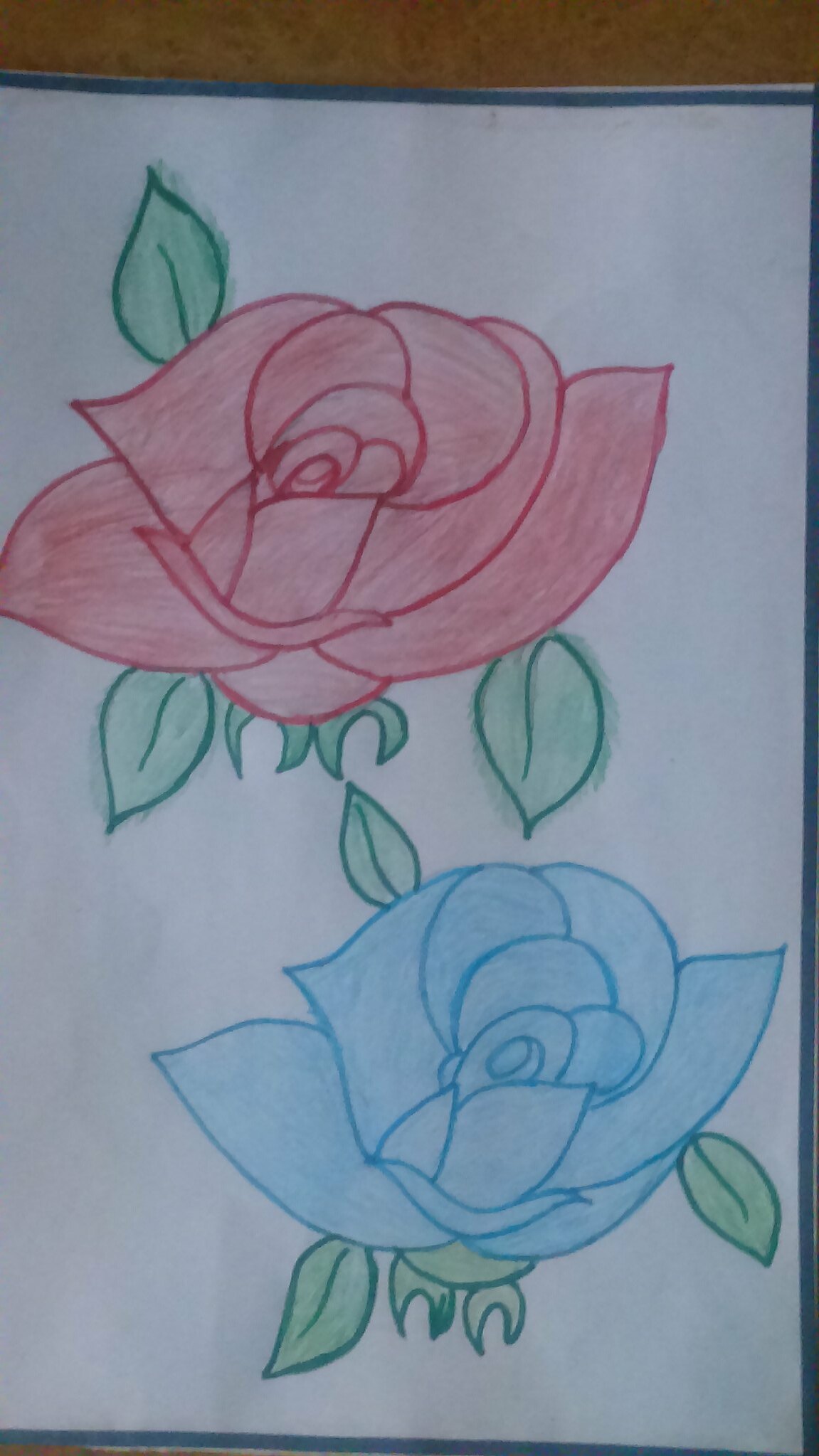The image captures a top-down view of a white piece of paper featuring two hand-drawn flowers. The flower at the top is oriented slightly to the left and depicts a red rose. This rose is outlined in darker red and shaded with lighter red, complemented by three teardrop-shaped leaves, each outlined in darker green and filled with lighter green shading. At the bottom right of the paper, there is another flower in a similar style, but in blue. This blue flower is outlined in a darker blue and filled with a lighter blue, also accompanied by three teardrop-shaped leaves, outlined and shaded with varying hues of green. Both flowers exhibit delicate and meticulous hand-drawn details, illustrating a harmonious blend of colors and precise petal and leaf shapes.